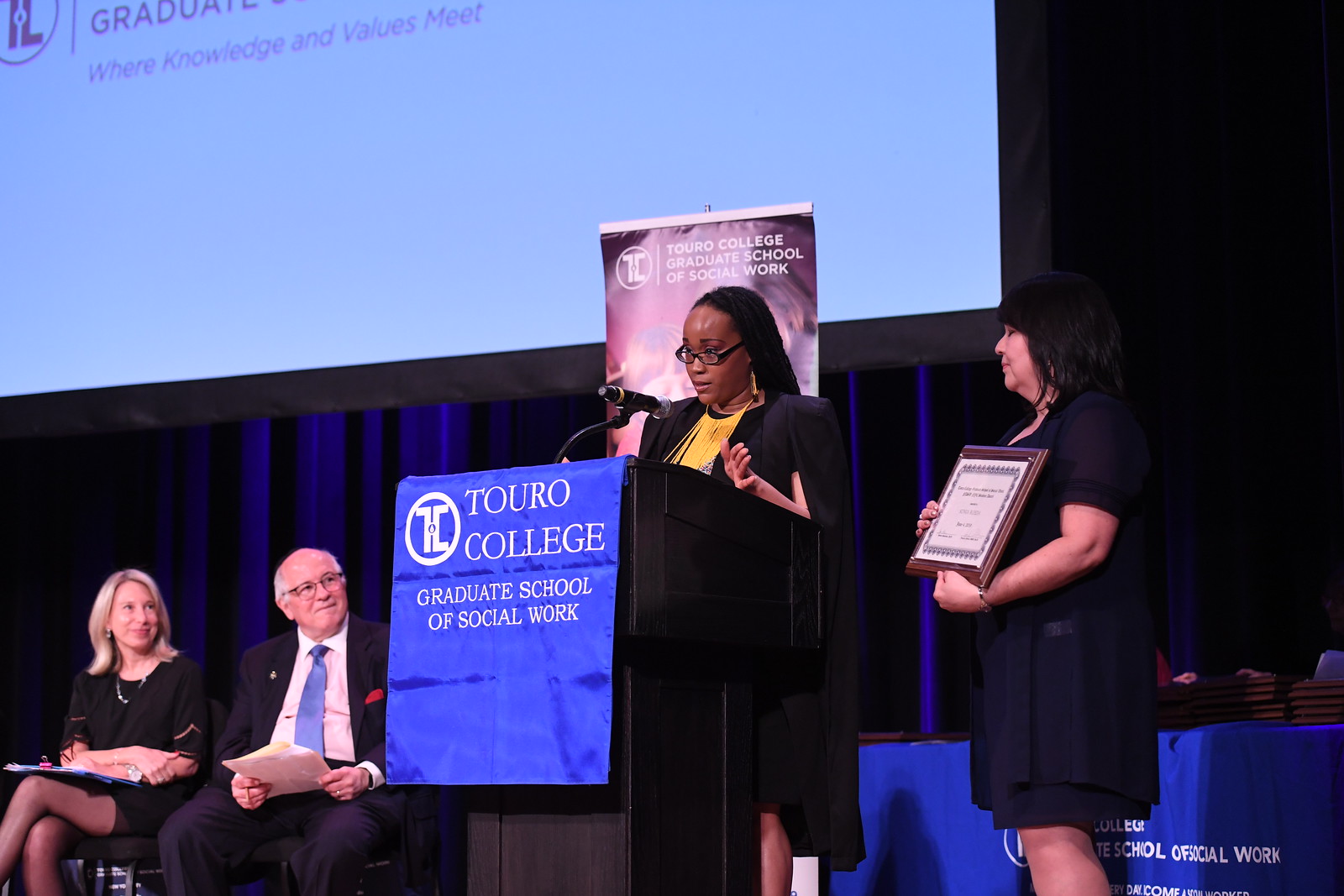In this detailed photograph, a moment of academic achievement is vividly captured on an indoor stage adorned with blue curtains. Central to the scene is a dark wooden podium draped with a blue banner reading "Touro College, Graduate School of Social Work." A woman with long braids, black-rimmed glasses, and a black dress complemented by a yellow blouse and necklace, stands behind the podium speaking into a microphone. To her right, a young white woman with dark hair, dressed in a long dark dress, proudly holds her graduation certificate, signifying her completion of a graduate degree, likely a master's from the Graduate School of Social Work.

To the left of the podium, two individuals observe the ceremony. Seated on chairs are an older white man with gray hair and eyeglasses, dressed in a black suit with a blue tie, holding papers, and a white woman with blonde hair clad in a black dress, with a clipboard resting on her lap. Both are intent on the speech being delivered. A large projector screen and a poster with text provide a backdrop to this inspiring scene of academic accomplishment.